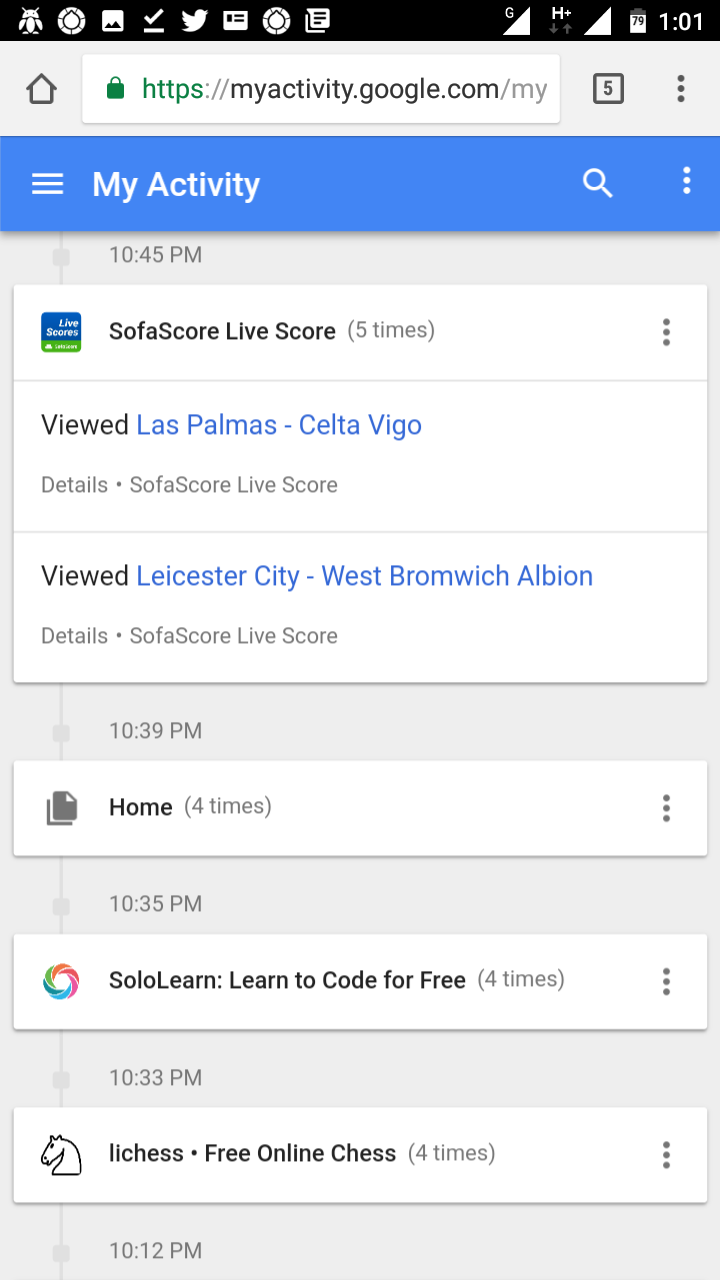A person is viewing their activity history on their smartphone through the website MyActivity.Google.com. The header of the page clearly shows the title “My Activity.” The screen displays a detailed log of the user's recent interactions across various Google services for a specific date, listed in descending order of time. The most recent activity at 10:45 PM shows a visit to SOFA Score to view live scores, specifically for a match between Las Palmas and Celta Vigo. The next recorded activity, at 10:39 PM, is a visit to Home Score Times. At 10:35 PM, the user accessed SoloLearn, a platform for learning to code for free. This is followed by an activity logged at 10:33 PM, which indicates that the user visited Lichess, a free online chess platform. The background of the page is predominantly white or gray, with occasional blue accents, giving it a clean and simple appearance. This detailed log highlights how Google tracks user activities across different platforms and services while logged into their Google profile.